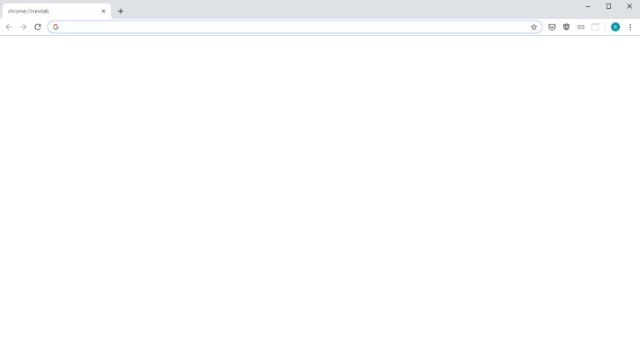The screenshot depicts a completely blank, white screen within a Google Chrome browser window. In the upper left corner, there is a partially visible tab labeled "Chrome" followed by an indistinguishable, blurry word. Adjacent to this tab, there is a dark gray plus (+) symbol for adding new tabs. On the opposite side, in the upper right corner, the standard browser window controls for minimize, maximize, and close are visible.

Directly beneath the tab area, navigation icons such as the grayed-out forward and backward arrows are present, indicating that no browsing history is available. To their right, the reload symbol is also visible. The URL bar is empty, showing no web address, and the only visible elements are a Google icon on the left and an option to add a favorite on the right. Further to the right, in the top corner, a green icon signifies that a user is signed into Google Chrome. Next to this, the three vertical dots are present, indicating a menu that can be accessed for additional browser options. 

Overall, the image captures the initial, unaltered state of a new Chrome browser tab, poised for user interaction.